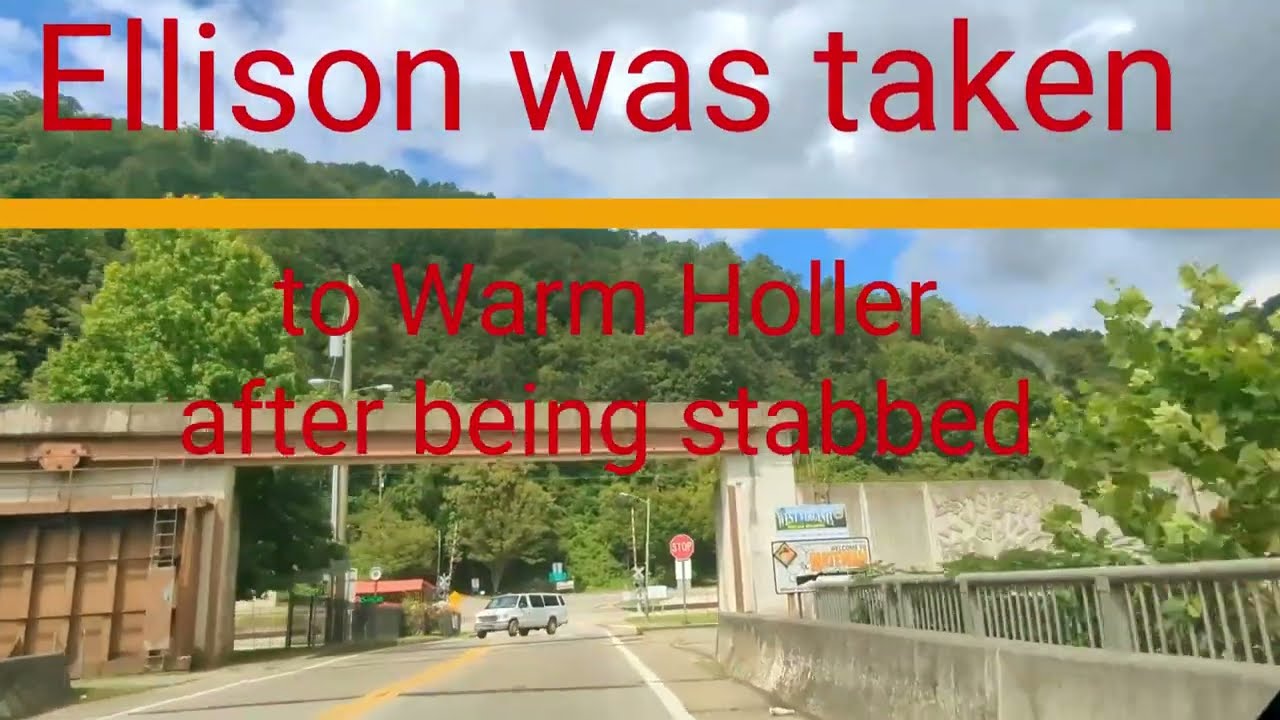The image captures a vivid scene of a forested area during a warm, slightly overcast day, with lush green leaves in full bloom under a hazy sky. Dominating the foreground is a bridge, likely an overpass, characterized by its concrete barriers and guardrails. Below this structure, a white van can be seen traveling on a road, heading towards a checkpoint marked by a stop sign and a small building with a rounded wall section and a ladder leading to a small ridge or overhead pillar. Prominently displayed in red text across the photo is the message: "Ellison was taken to Warm Holler after being stabbed," followed by an orange stripe. Additional signage includes a white sign with an unreadable smaller text and arrows, hinting at directions or specific locations, as well as a railroad crossing sign and barriers. The scene appears to be related to a crime, suggested by the text overlay and the detailed descriptions of the setting.